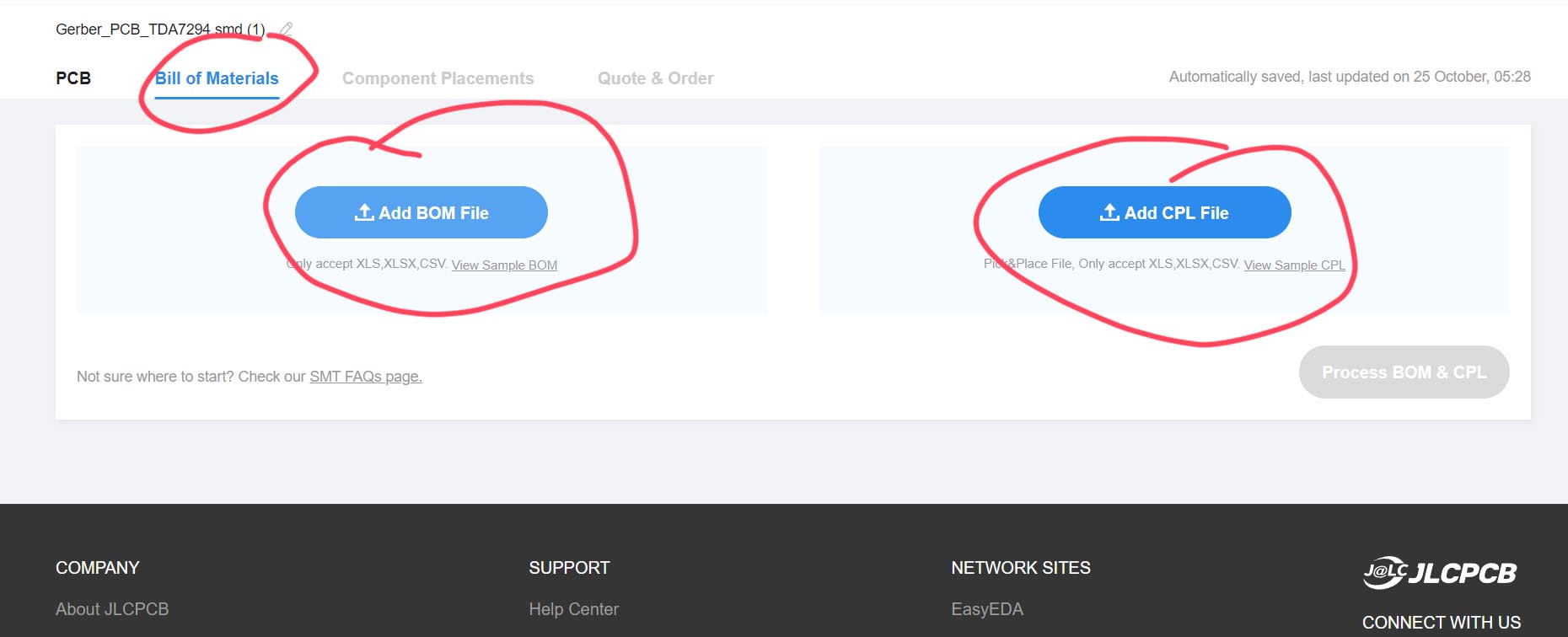This image is a detailed screenshot captured from a website's user interface. At the bottom of the page, there is a sleek black banner with various sections listed in white text. On the left, it reads "Company" followed by "About JLCPCB." Next, the section titled "Support" is followed by "Help Center." "Network Sites" comes next with "EZEDA" listed beneath it. Further right, it says "J at LC" and then "JLCPCB," followed by a call to "Connect with Us."

At the top of the page, a white background features the file name "Gerber_PCB_DDA_7294_SMD (1)" with a pencil icon next to it. Below this, the text "PCB" appears, followed by "Bill of Materials" in blue text with a red circle around it. Other sections include "Component Placements" and "Quote and Order." 

On the right-hand side, it indicates "Automatically saved, last updated on October 25 at 05:28." Below this timestamp, the layout divides into two main panels. The left panel has instructions to "Add BOM File" with an upload button circled in red. Adjacent to this is another option to "Add CPL File," also highlighted with a red circle. Lastly, the phrase "Process BOM and CPL" is visible. On the extreme left, there is guidance reading, "Not sure where to start? Check out our SMT_FAQs page."